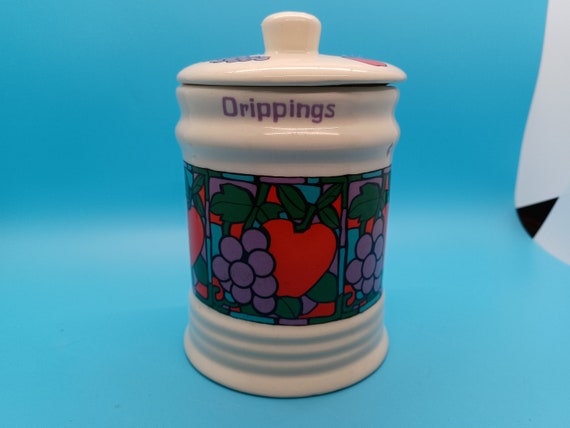The image depicts a white ceramic drippings container set against a bright blue background, which appears to be a folded piece of paper. The lid of the container features a simple handle and is decorated with a painted design—grapes to the left and an apple to the right. Below the lid, it says "drippings" in purple text. Around the middle of the container, there is a recurring pattern with illustrations of grapes and apples, reminiscent of a stained glass style, framed by a border of red, blue, and purple. Each section of this pattern is contained within a square shape that repeats horizontally around the jar. The background also shows signs of curling, suggesting it’s part of a makeshift or product photography setup. The container has three ridges near the bottom, adding to its ornate design. In the background, aside from the blue paper, a hint of a white wall and some obscured objects can be seen.